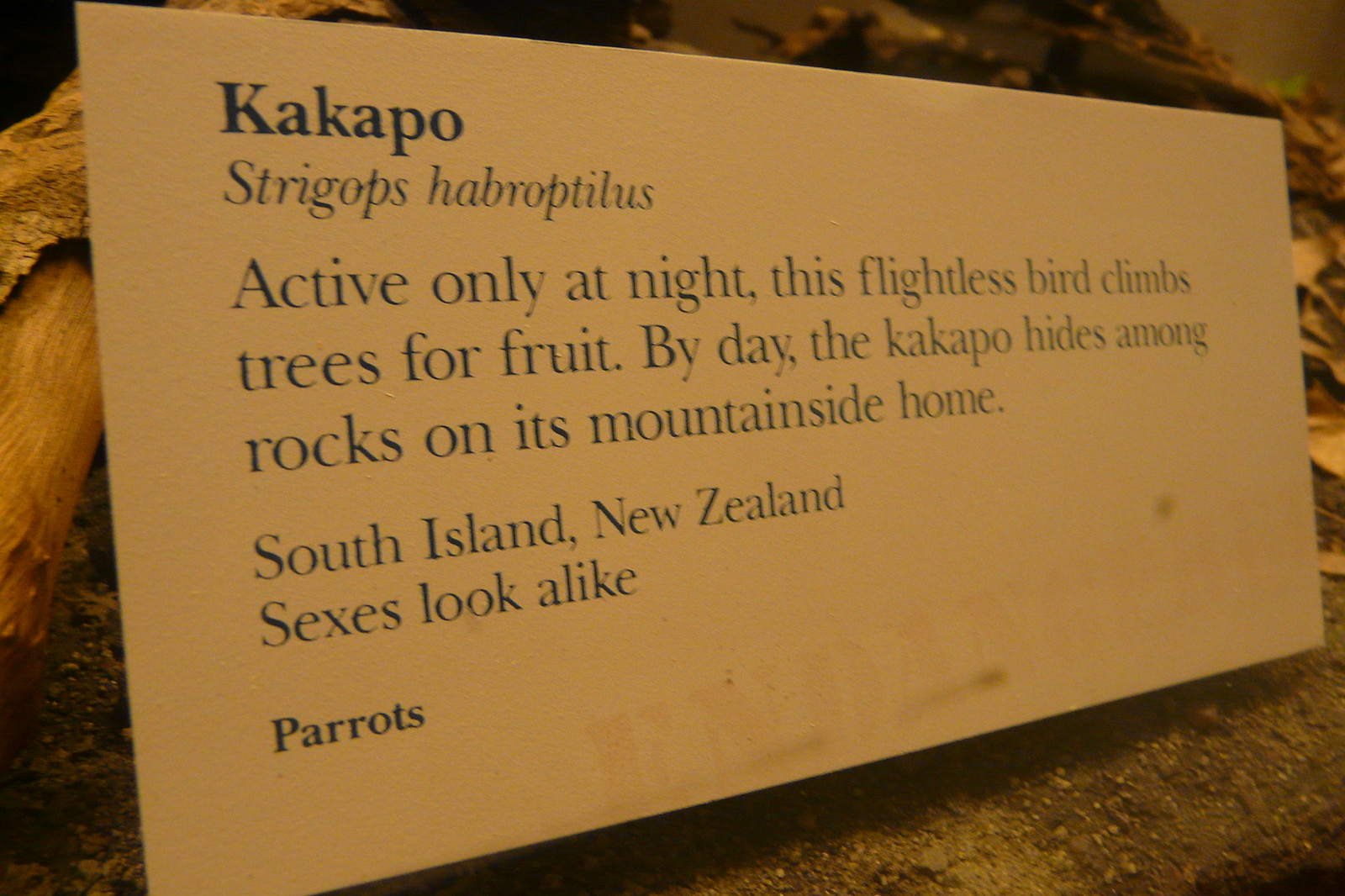This image features a horizontally rectangular informational sign about the Kakapo bird, located likely outside a zoo exhibit or museum display. The sign is distinct with its white background, adorned with bold black lettering. The card appears to be mounted on or beside a wooden surface, with dirt visible underneath.

At the very top of the sign, "Kakapo" (K-A-K-A-P-O) is prominently displayed, followed by its scientific name, "Strigops habroptilis." The text describes the Kakapo's behavior: "Active only at night, this flightless bird climbs trees for fruit. By day, the Kakapo hides among rocks on its mountainous home in the South Island, New Zealand." Additional details note that the sexes look alike. At the bottom, the word "Parrots" is written in slightly smaller but bold font, indicating that the Kakapo belongs to the parrot family.

Overall, the card is a clean and informative snapshot of this unique bird's habits and habitat, emphasizing its nocturnal nature, flightlessness, and location in New Zealand.